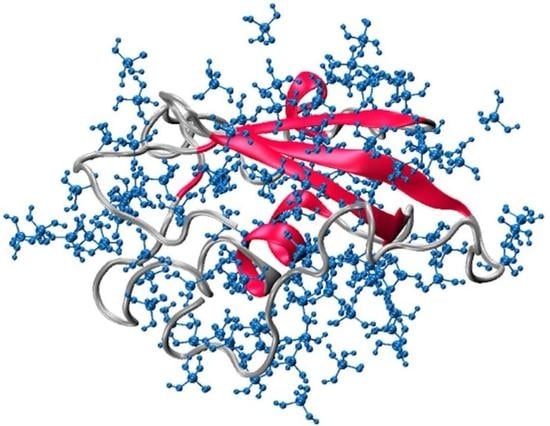This abstract image features an intricate network of blue, holly berry-like cells interconnected by gray lines, resembling molecular structures. Each cluster contains approximately 8 to 10 blue circles that form complex, web-like patterns. Dominating the white backdrop is a pink, ribbon-like element sprawling and curling throughout the composition, intertwining seamlessly with the blue cells. Additional silver streamer-like cords emanate from the red ribbon, weaving above, below, and around the central elements, adding to the overall complexity. The combined effect is a detailed, DNA-like portrayal that merges organic and abstract art, showcasing a delicate interplay of blue, gray, and pink hues.